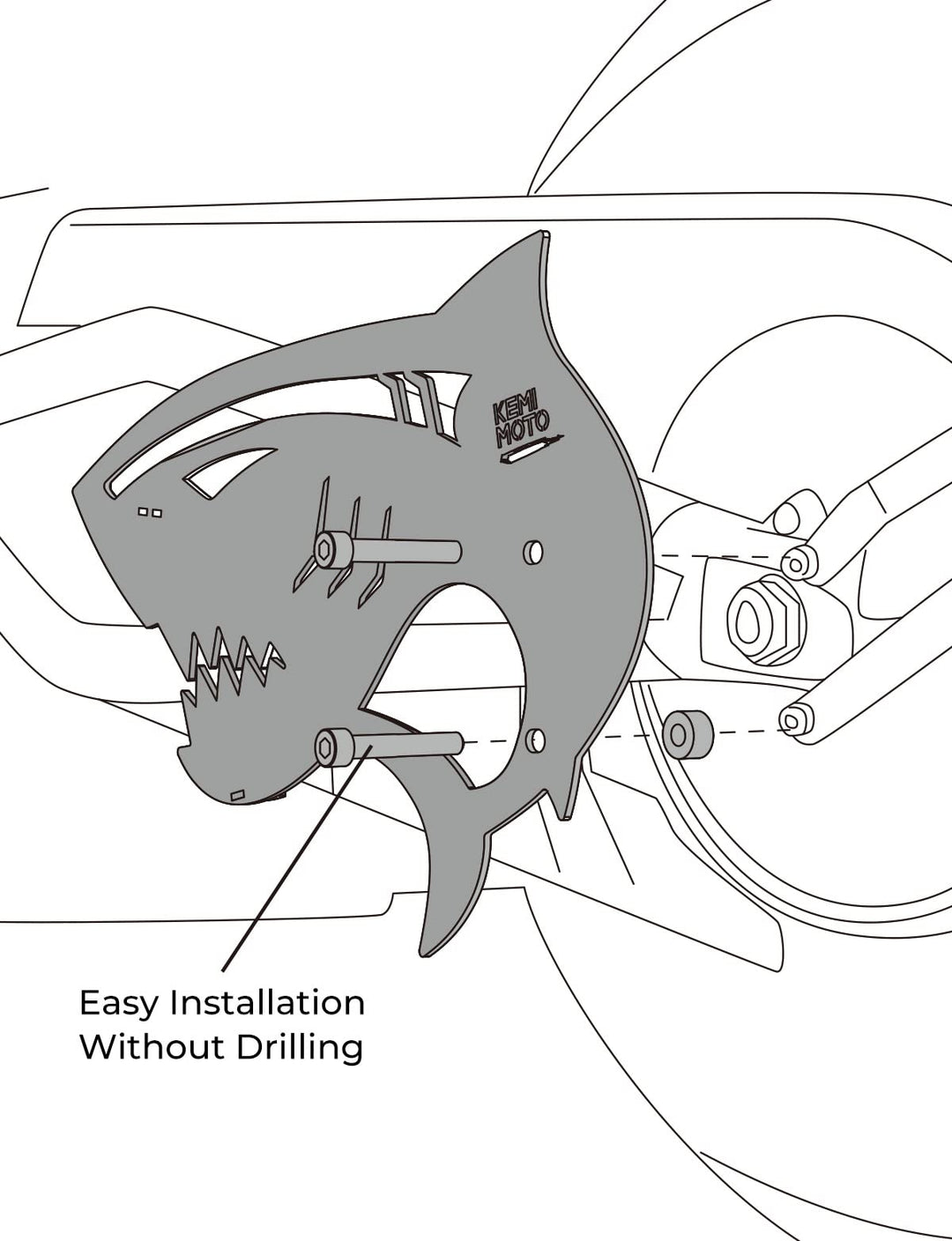This is a detailed black and white illustrated diagram for the easy installation of a metallic plate, which appears to attach to a motorcycle or car wheel without the need for drilling. The image prominently features the part shaped like a ferocious animal head, interpreted by different viewers as either a shark, leopard, lion, or an angry cat, complete with jagged teeth forming the mouth. The plate's design includes cutouts resembling eyes and gills, enhancing its animalistic appearance. Two screws are depicted, showing where they are to be inserted to secure the plate to the vehicle. The background includes various lines, nuts, bolts, and metal hinges, hinting at the complexity of the connected mechanical components. "K-E-M-M-O-T-O" is labeled on the part, and the phrase "easy installation without drilling" is clearly marked at the bottom of the diagram. Additionally, a tire shape is faintly visible in the background, indicating the plate's placement in relation to the vehicle's wheel.